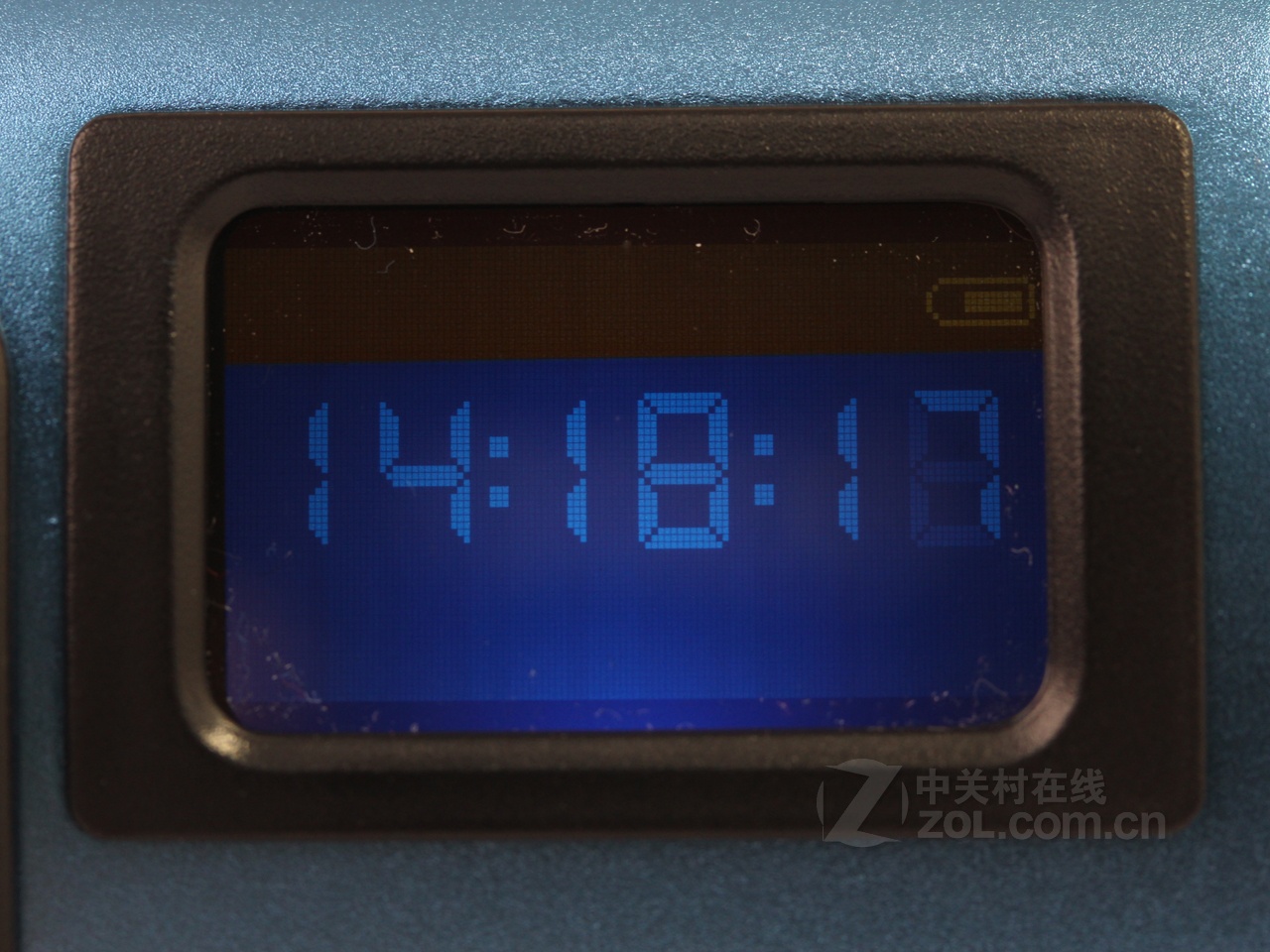This close-up photograph features a digital clock embedded within a larger piece of medium-light blue, grainy-textured vinyl. The clock is framed by a sleek, black rectangular vinyl casing. The clock's display has a blue face with light blue, illuminated numbers, showing the time as 14:18:17. In the bottom right corner of the clock screen, a capital letter 'Z' accompanied by Asian characters can be seen, followed by the web address "zol.com.cn" beneath the characters.